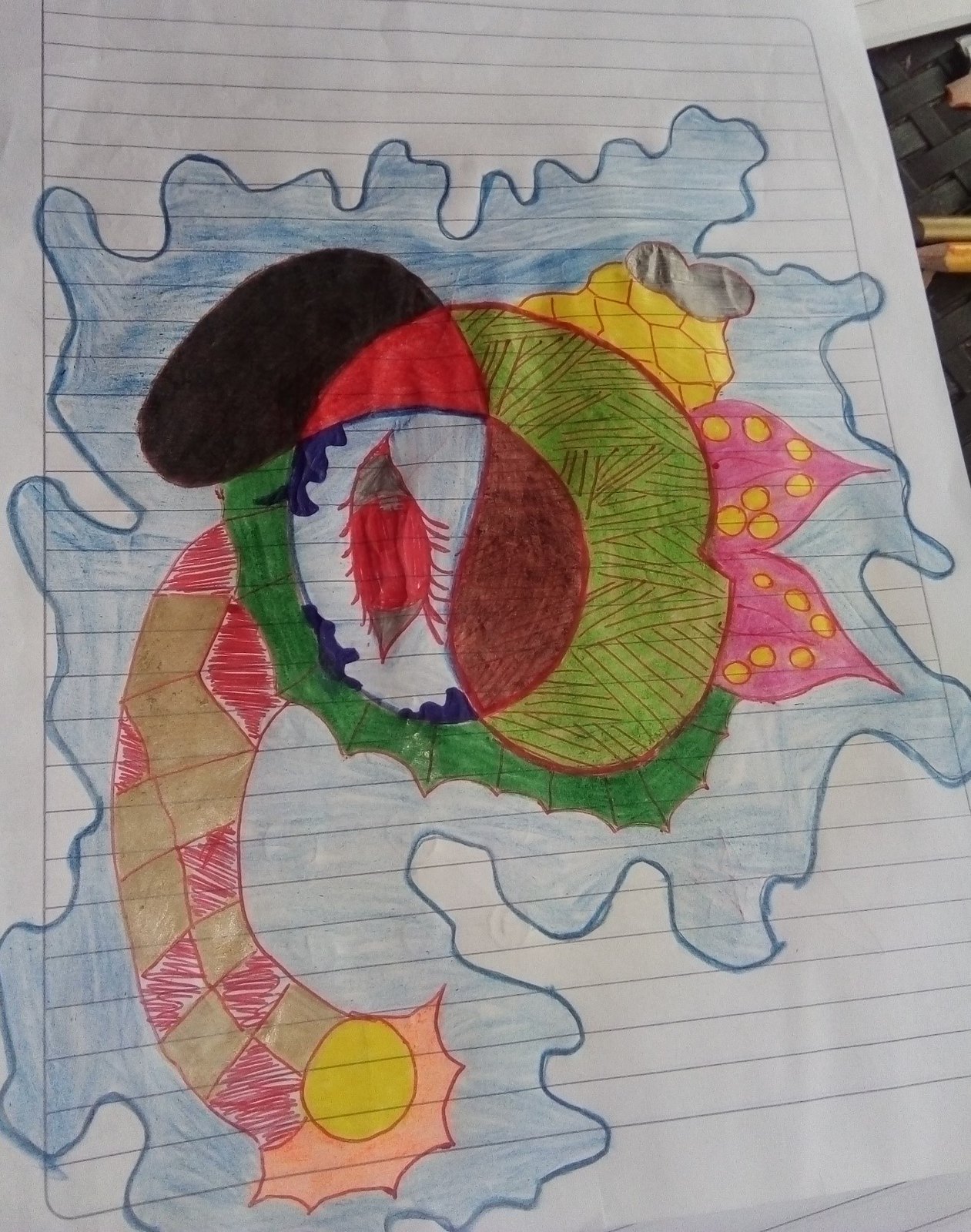The photograph features a piece of white A4 lined paper, commonly found in a school notebook, with various doodles possibly done during a moment of boredom. The lined paper has a distinct gray line pattern with a solid white border. The central element of the drawing is a large, amoeba-like shape outlined in dark blue and filled with a lighter blue color. Within this blue shape, there are multiple smaller, colorful shapes and designs.

To the side, there is an intricate drawing of an eye that is red with brown edges, surrounded by a white area and a navy blue outline. Nearby, a yellow shape with a red outline resembles a honeycomb design, overlaid by a gray peanut shape. Pink shapes, potentially resembling pomegranates with yellow seeds, are also present. Additionally, there is a section of light green with red outlines and lines, and various other randomly scattered shapes in hues of red, black, and brown.

Extending from the blue shape is a handle-like form that is checkered with red and brown shades. At one end of this handle is a starburst-like figure colored in red with a yellow circle at its center, akin to a sun shape. Throughout the doodle, diverse shapes, colors, and textures — including ones that appear to be an elephant's trunk, a leaf, and almond shapes — collaborate to create a visually engaging, multifaceted piece of artwork.